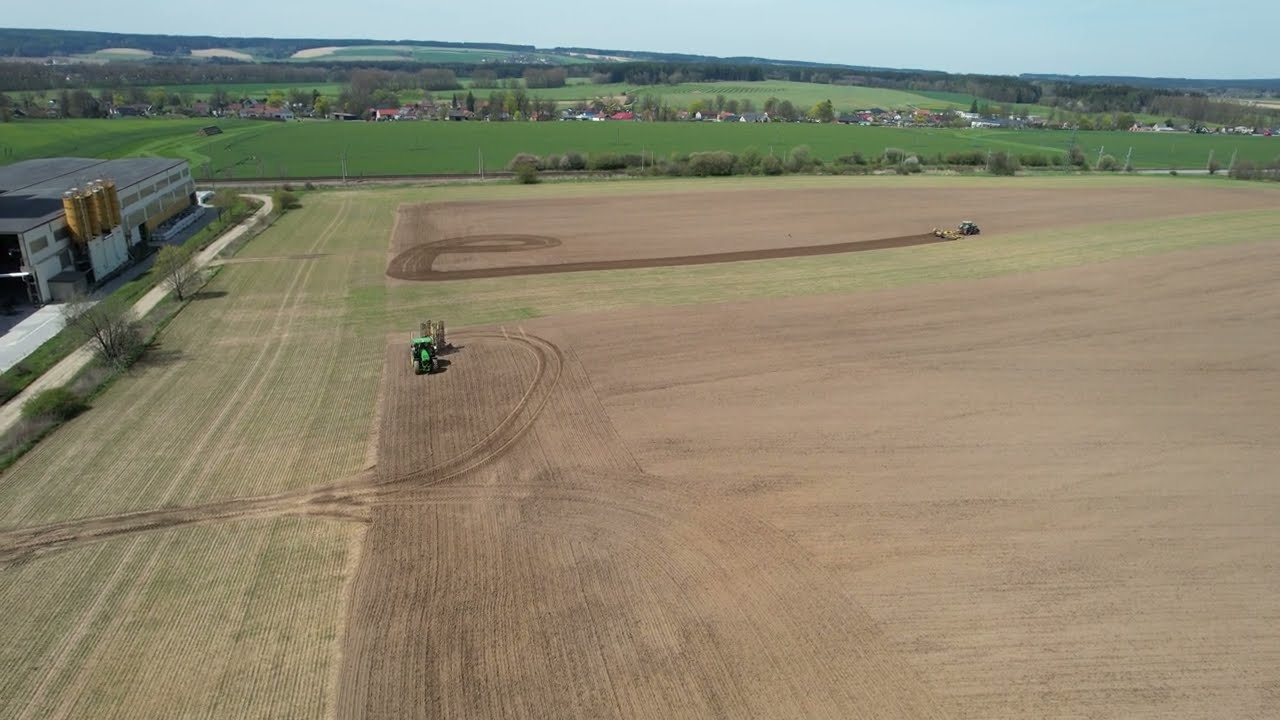This color aerial photograph, likely taken from a drone or plane, captures a vibrant farmland under a bright blue sky. Dominating the forefront is a vast greenish-brown field with noticeable dirt tracks created by two active tractors; one tractor moves right, while the other heads forward. Toward the left, there’s a cluster of commercial buildings resembling storage barns, surrounded by a walkway. Adjacent to these structures, a stretch of green grass contrasts with the predominantly brown, plowed soil. The background reveals expansive verdant pastures and a hilly landscape dotted with numerous houses and trees, extending into the distance under the light blue sky. The overall image conveys a sense of idyllic agricultural activity amidst a picturesque rural setting.